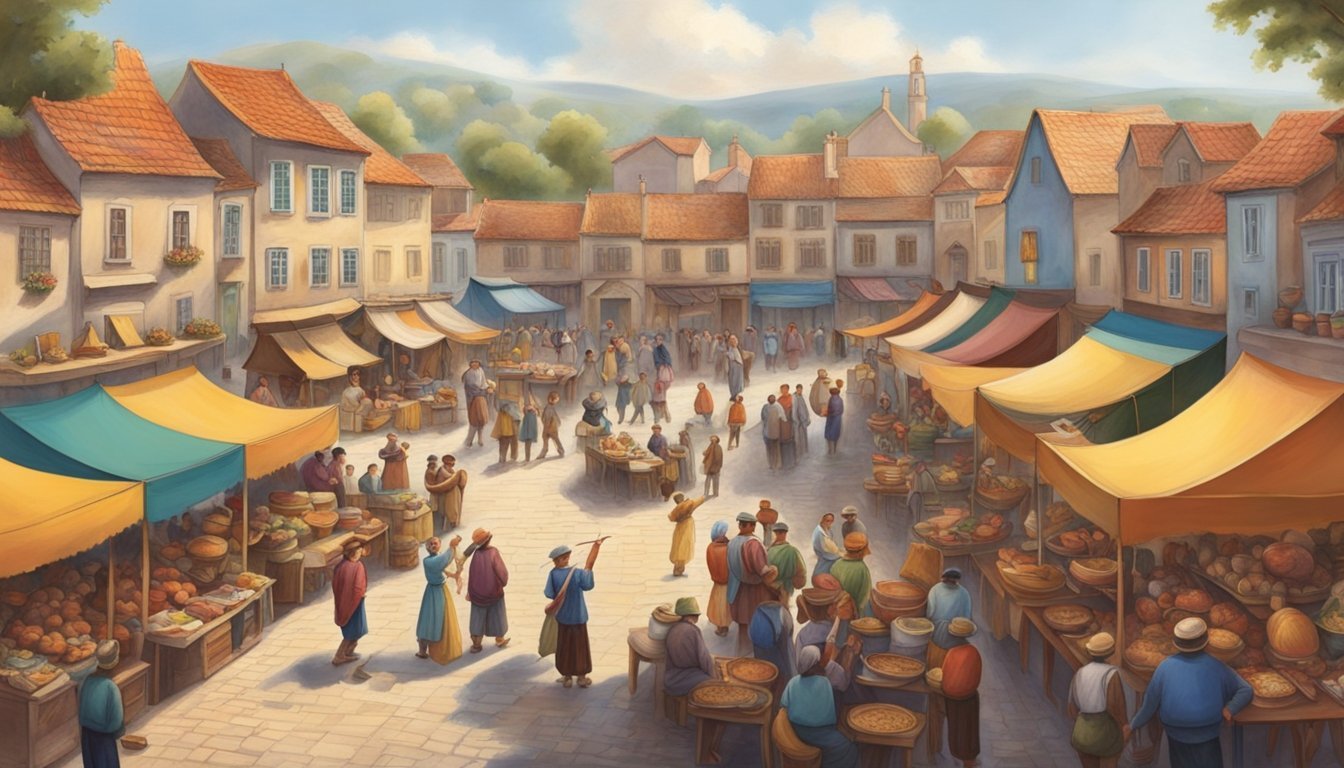This painting depicts a bustling early 1900s town square marketplace set against a vivid backdrop of blue skies with puffy clouds, rolling hills, and green trees. The marketplace is surrounded by a semi-circle of two-story white buildings with orange roofs, which house various stores and businesses. In front of these structures, numerous booths with blue and yellow awnings display an array of goods. The light grey and white cobblestone ground adds to the charm of the scene, where townsfolk in colorful outfits browse the assorted wares. Among the bustling market stalls, one can see loaves of bread, bakery items, vegetables, citrus fruits, and even pizzas being offered to eager shoppers. The vibrant activity and detailed setting create a vivid portrayal of community life in an era gone by.